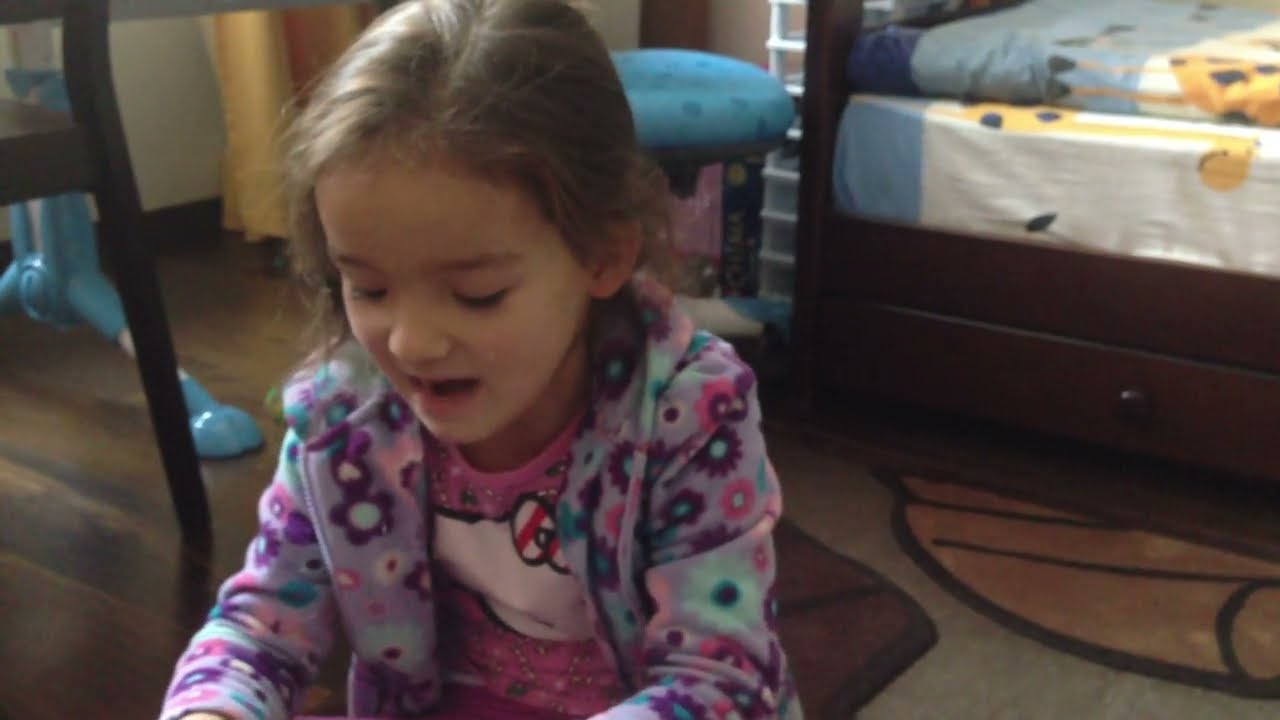In the color photograph, a young girl, around four or five years old with medium brown hair pulled back, sits on a light golden hardwood floor in her bedroom. The girl wears a pink Hello Kitty shirt underneath a purple fleece jacket adorned with purple, pink, and green flowers. Her gaze is directed downward, though what she is looking at is not visible in the crop of the photo. Scattered around her on the floor are a few toys. Behind her, there is a dark wood bed with a sheet patterned in gold-toned animals, and a blanket. A rug lies underneath the bed. The bedroom also features gold curtains hanging from a window behind her, a blue stool beside the bed, and a brown wooden chair with another blue object behind it. The photograph, taken in landscape orientation, captures the scene with a high degree of detail and realism.